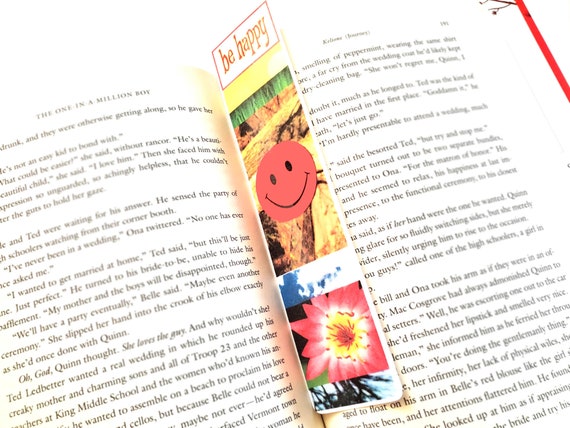This image captures an overhead view of an open book, titled "The One in a Million Boy." It is open to pages 190 and 191, revealing a passage which includes dialogue: "He's not an easy kid to bond with. What could be easier, she said, without rancor. He's a beautiful child, she said, I love him. Then she faced him with an expression so unguarded, so achingly helpless that he couldn't muster the guts to hold her gaze." The book is held open by a colorful bookmark adorned with a bright orange smiley face and a vibrant pink flower with a yellow center. At the top of the bookmark, red lettering reads "Be Happy." The pages of the book are angled so that its top right corner reaches the right side of the image, while the bottom left corner is cut off. The bookmark also features sections of nature-themed images, including grass, woods, clouds, and branches, though the happy face dominates its visual space. The book rests on an indeterminate white surface, with some of the bottom edges of the pages appearing whited out.